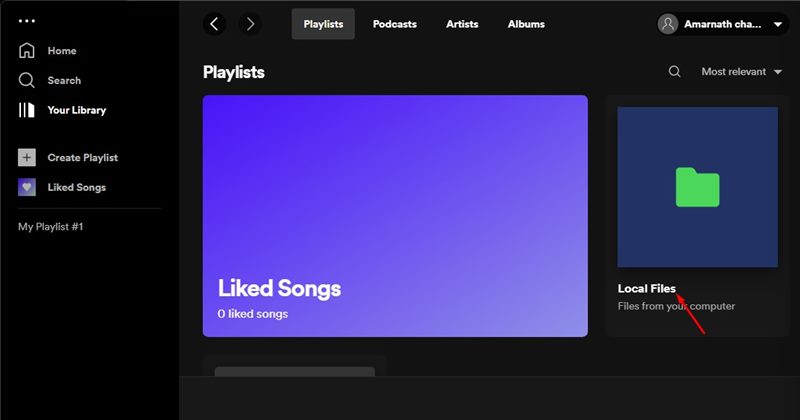The image depicts a webpage interface, primarily for a music streaming service. At the top, there are navigation arrows - a back arrow and a forward arrow. The interface includes tabs labeled "Playlists," "Podcasts," "Artists," and "Albums." In the top right corner, there is a username displayed alongside an icon outlined in grey. 

Below this section, prominently displayed against a bright purple background, is a label reading "Liked Songs" with a status indicating there are zero liked songs. Adjacent to this, a green folder icon on a blue background is labeled "Local Files," accompanied by the description "Files from your computer." A red arrow points towards the "Local Files" label for emphasis.

To the left side of the webpage, a vertical navigation menu lists several options. These include "Home" with a house icon, "Search" featuring a magnifying glass icon, "Your Library," "Create a Playlist" with a plus sign, and "Liked Songs" with a silver heart icon on a purple background. Below these options is "My Playlist #1."

The overall design employs a black background with grey text, while incorporating various vibrant colors for key elements, such as the bright purple for "Liked Songs" and the blue background for "Local Files."